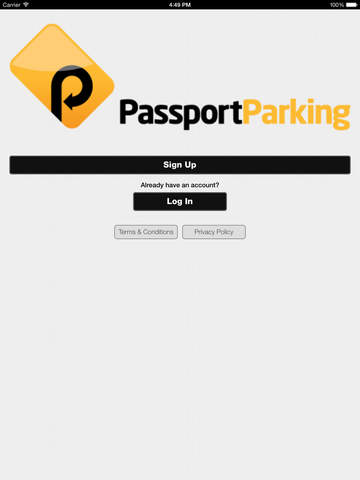The image depicts the home page of the Passport Parking website, prominently featuring its logo. The logo consists of a yellow, tilted rectangle with a black arrow integrated to form the letter "P," representing "Passport." The text "Passport Parking" is displayed below the logo, where "Passport" is written in black and "Parking" in yellow.

Directly beneath the logo and text, there is a long, thin black rectangle spanning the width of the screen, labeled "Sign Up" in white text. Below this, the phrase "Already have an account?" appears in black text, followed by a smaller black rectangle with the option to "Log In."

Two barely visible, grayish buttons are located further down the page, labeled "Terms and Conditions" and "Privacy Policy." The entire page has a plain, whiteish-gray background, lacking vibrant colors or exciting elements, designed simply for user login and registration.